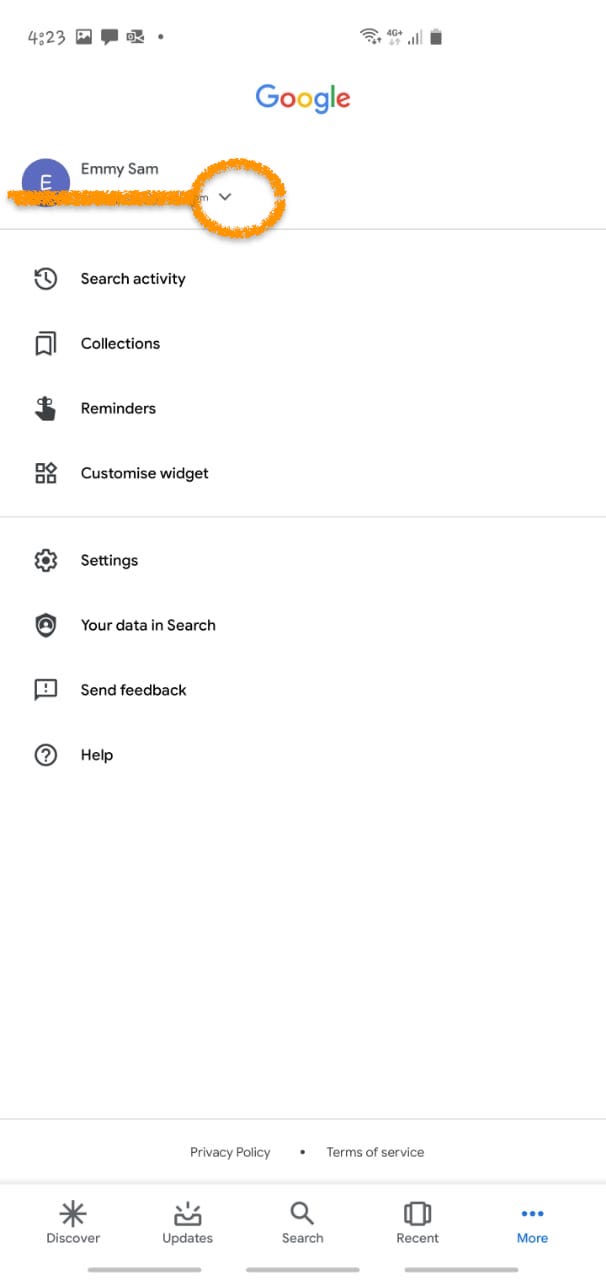In this image, we see a detailed screenshot of a Google account interface on a mobile device. At the top right corner, the battery icon displays approximately 90% charge, and next to it, the Wi-Fi signal strength is indicated with three filled bars out of four. Further to the left, the status bar shows "4G+" for mobile network connectivity, and at the top left, the time is 4:23 PM. On the top right corner, there are three icons: a picture icon, a chat bubble, and an envelope, which likely represent notifications or messages.

Dominating the top center of the image is the Google logo, featuring its iconic colors: blue, red, yellow, blue, green, and red. Below this is the account information, where the name "Emmy Sam" is prominently displayed. To the left of the name, there is a blue circle avatar with a white interior. The email address associated with the account is obscured by an orange line for privacy, and an orange circled dropdown arrow is located to the right of this line, indicating additional account options.

Beneath the account information, a list of categories is organized vertically. These categories include: Search Activity, Collections, Reminders, Customize Widgets, Settings, Your Data in Search, Send Feedback, and Help. Each category likely provides access to different aspects of the user's Google account settings and data management tools.